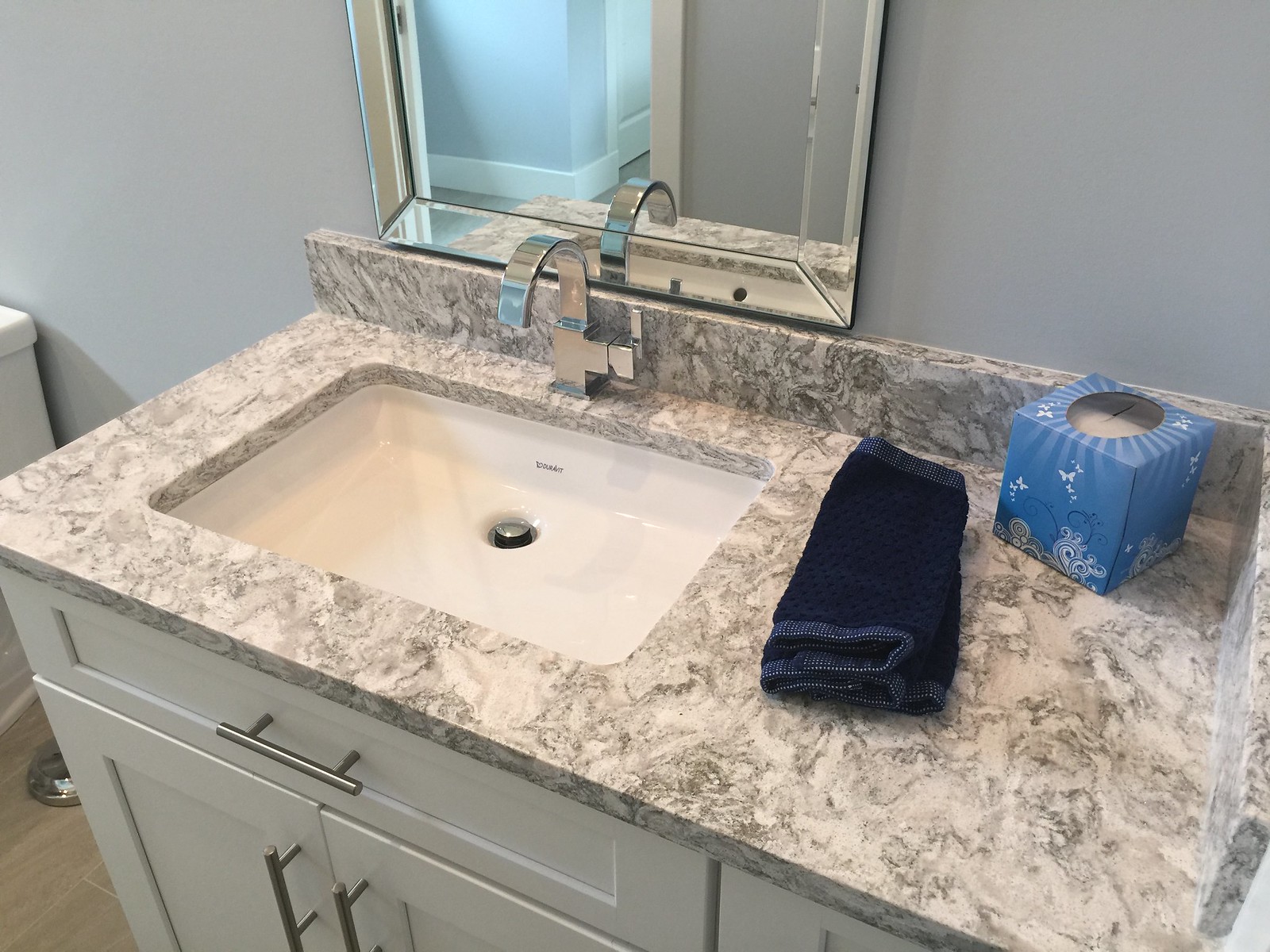The photograph showcases a modern bathroom vanity featuring a faux marble countertop with a square basin and a sleek silver faucet. Positioned just above the splash guard is a mirror, reflecting the clean aesthetic of the space. To the side of the basin lies a dark blue or deep purple washcloth, neatly placed next to a full, unopened box of tissues, which displays a charming sea creature motif. Below the countertop, the vanity includes two white drawers adorned with antique brass handles, along with cabinet doors underneath the sink. In the background, the edge of a toilet is visible, completing the glimpse into this well-appointed bathroom.